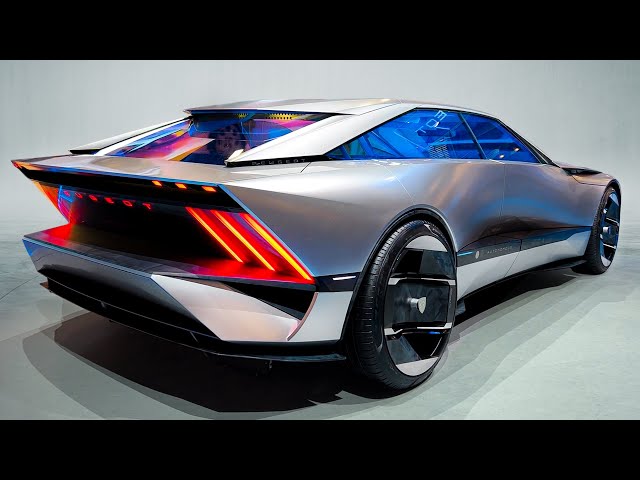The image depicts a highly futuristic, expensive sports car set against a grey background. The car features a sleek, fluid, and aerodynamic design with a metallic chrome color that reflects surrounding lights dramatically. It is a two-door model, and the lack of visible door handles adds to its futuristic appeal. The windows have a distinct blue tint, while the small rear window is multicolored. Notably, the car has unique, unconventional wheels that deviate from the traditional spoke design, enhancing its avant-garde appearance.

At the rear, the car boasts a subtle spoiler above a black bumper, and its taillights, located between the spoiler and bumper, glow brilliantly in red and yellow hues. Additional yellow lights are positioned above the brake lights, contributing to the car's high-tech look. Shadows and reflections are visible around the car, adding depth to the image and further emphasizing its modernity. Overall, this car exudes a sense of luxury and cutting-edge technology, standing out as an extraordinary piece of automotive design.